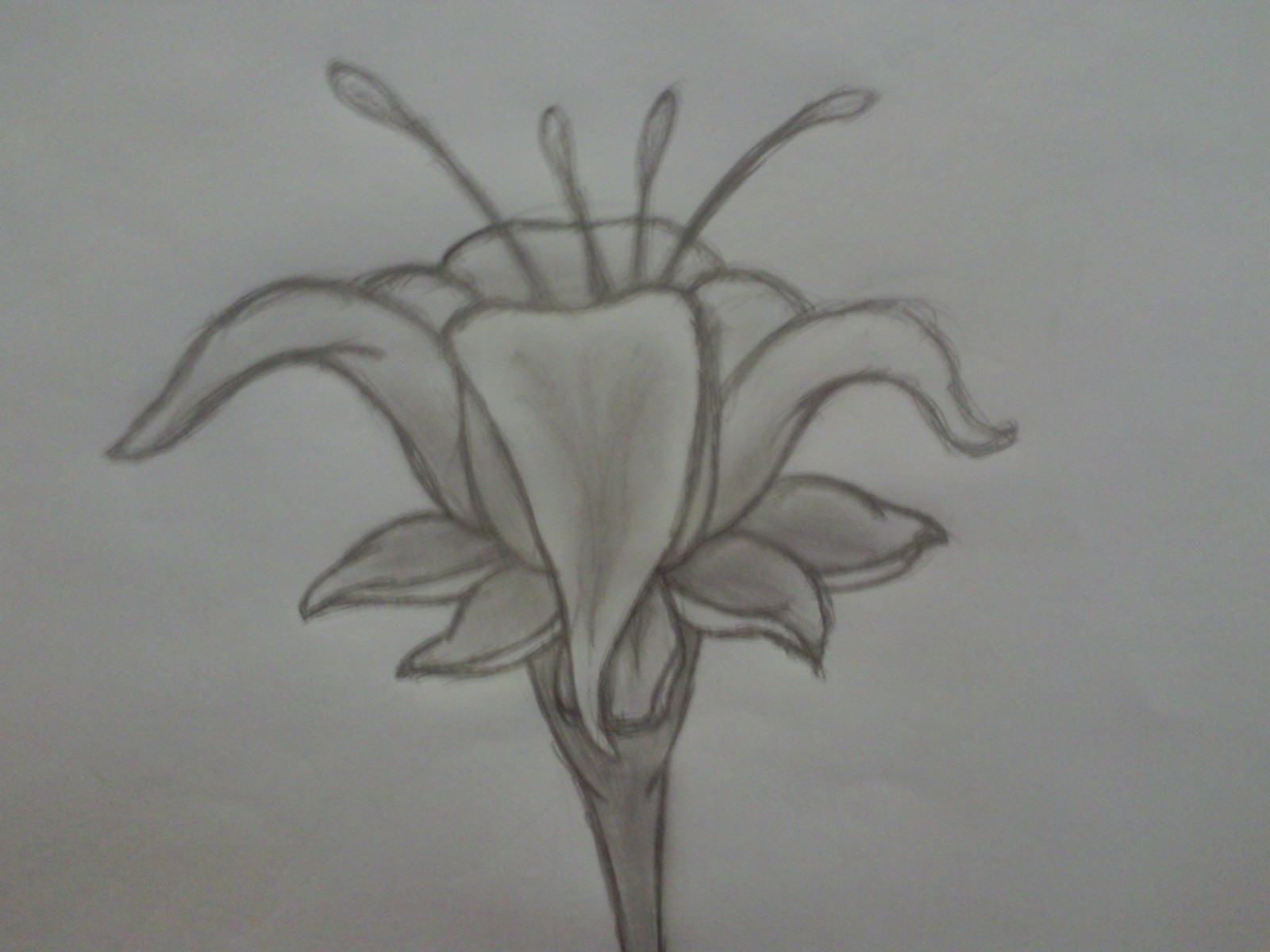This image depicts an intricate illustration of a flower rendered in either pencil or charcoal, showcasing a textured, monochromatic appearance. The flower’s outline is meticulously drawn, highlighting multiple elongated petals that boast graceful curves, arching upwards from the center and gently curving downward. Some petals have a delicate wave at their ends, and there appear to be about six of them in total.

The flower's core features tiny, slender stems adorned with small, rounded tips, numbering four. At the base of the bloom, there are several finely detailed leaves, with around five visible on one side. This intricate portrayal extends to a darker-shaded stem that contrasts with the lighter blossoms, all set against the stark white background of the paper.